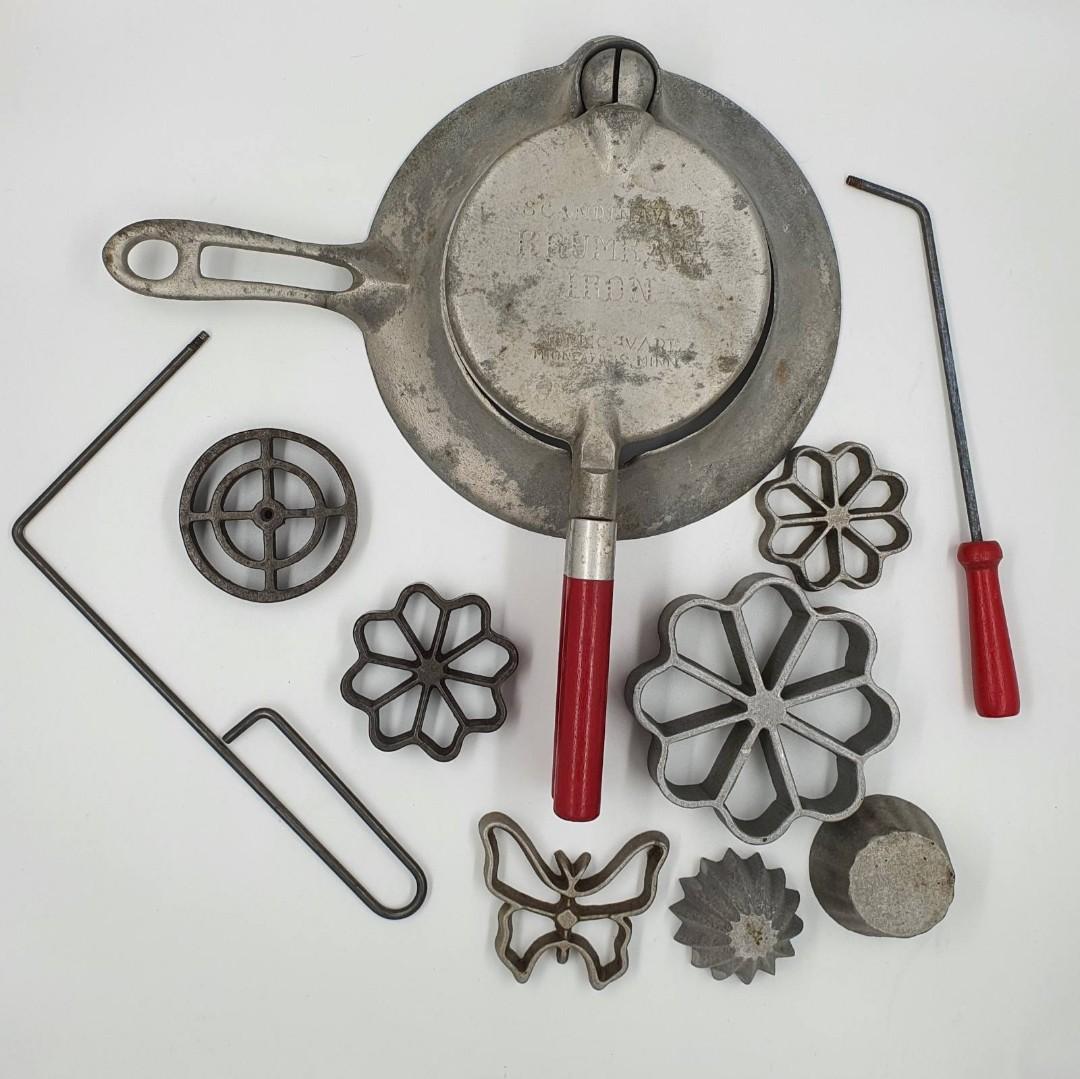This detailed photograph showcases a collection of unique metal cast items, possibly crafted by a past artisan, displayed against a solid white to grayish gradient background. The items, made primarily of cast iron, are arranged centrally to highlight their artistic quality. Among these creations, notable pieces include several metal snowflake-like designs, a butterfly figurine, and a spherical grill resembling a stovetop grate. There's a distinctive skillet pan with a long, red handle, accompanied by a fused, unique design that could be used for pressing pancakes. Another prominent feature is a large tool with a red handle, potentially used for lifting plates on a metal stove, hinting at its older, industrial nature. This tool, with engraved markings, is surrounded by various objects that resemble floral patterns, wedges, and two items akin to gear mechanisms or citrus juicers. Additionally, a couple of allen wrenches, one with a red handle and the other with a wire handle, add to the assortment of this meticulously crafted collection.